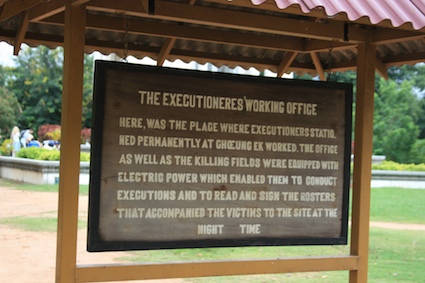The image depicts a detailed outdoor historical sign, mounted on a brown metal frame with a pink sheet metal roof. The frame consists of two vertical posts connected by horizontal bars at the top and bottom. Hanging from this frame, chains support a large rectangular wooden sign, painted brown with a dark brown border. In white lettering, the sign reads "The Executioner's Working Office," though "Executioner's" is misspelled as "Executioner'es." Below, it details: "Here was the place where executioners stationed permanently at Chekwang Eck worked. The office as well as the killing fields were equipped with electric power which enabled to conduct executions and to read and sign the rosters that accompanied the victims to the site at nighttime." The background reveals a lush, green setting with grass and trees, indicating the sign is located in what appears to be a public garden. The photograph is taken outdoor during the daytime, with clear, bright natural lighting enhancing the vivid colors and overall clarity of the image.